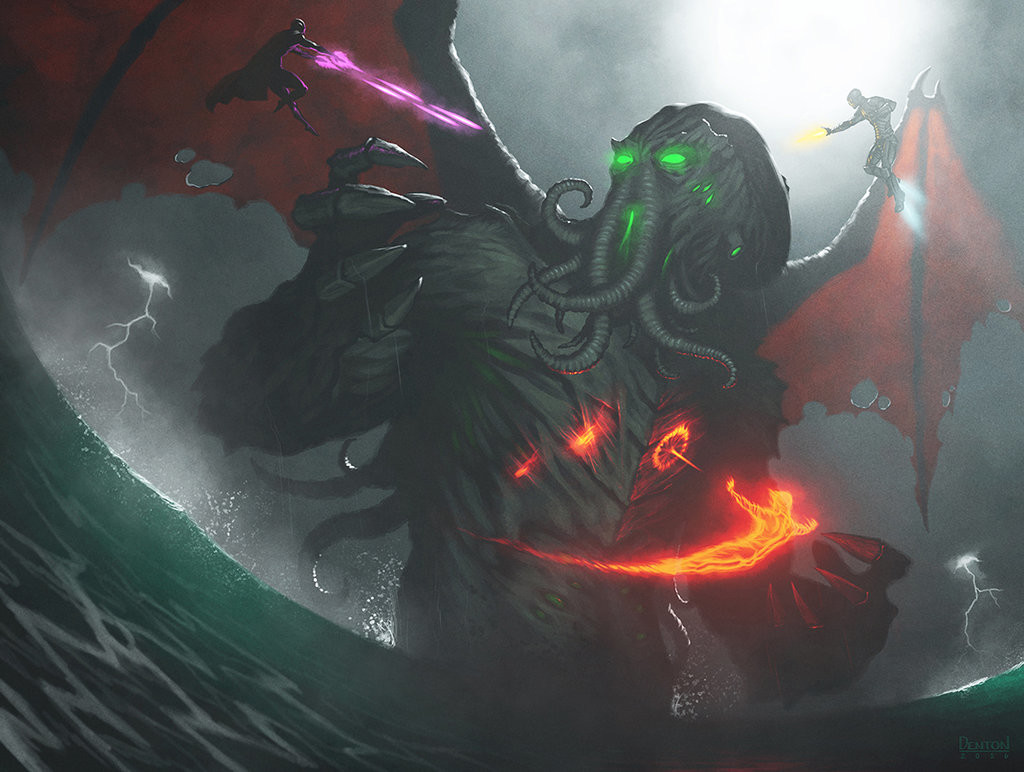A dramatic digital artwork captures a chilling scene of an epic battle against an eldritch monstrosity, reminiscent of Cthulhu. The image, cloaked in dark tones, showcases a monstrous creature emerging from a tempestuous ocean. Its tentacle-like appendages thrash menacingly, and its eerie green eyes glow ominously against its dark gray body and head. The creature's thick, grayish claws, tipped with long, pointed nails, reach menacingly towards its attackers.

Three valiant superheroes mount a desperate defense against the beast. In the top left, a caped figure unleashes purple energy beams, while another hero on the right fires yellow beams, his feet engulfed in blue flames. At the forefront, a being of pure fire directs a torrent of flames towards the monster. The ocean waves curve tumultuously to the left, almost forming a tsunami, accentuating the chaos of the storm. Lightning bolts tear through the stormy sky, illuminating the creature's immense, tattered red wings, which are outstretched in a terrifying display.